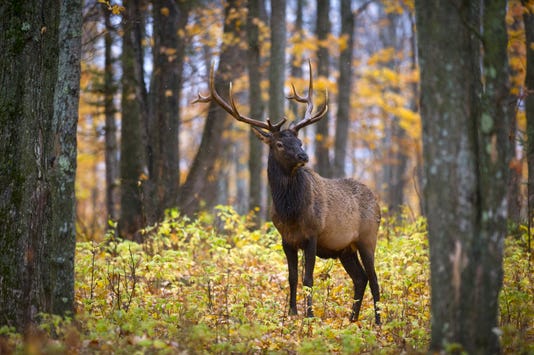In the heart of a forest, a majestic male elk stands regally, embodying the essence of autumn. Dominating the center of the image, the elk is poised on a lush forest floor adorned with tall, green plants and bathed in golden hues, signaling the fall season. The elk's impressive rack of antlers, with numerous branches, crowns his dark brown head and chest, which contrasts with his lighter brown body and dark brown legs. The elk's piercing gaze is directed slightly to the right, his ears alert and upright.

Surrounding the stately creature, the forest comprises tall gray-trunked trees, which frame the scene and stand vigil on either side. In the distance, the canopy of trees bursts into shades of yellow and gold, capturing the autumnal vibe. Slivers of blue sky peek through the dense foliage, adding a touch of serenity to the scene. The bark of the trees in the foreground provides a textured backdrop to this serene yet powerful woodland portrait, portrayed in photographic realism.